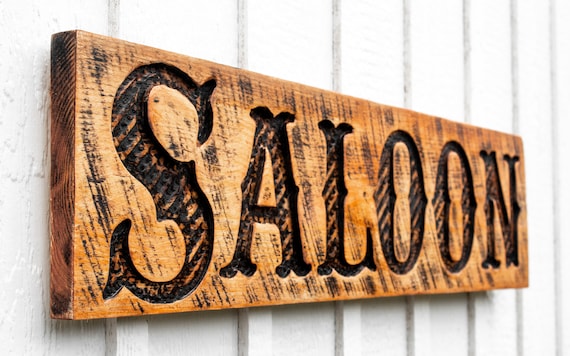The image features a photograph of a wooden sign that is prominently mounted on a white wooden wall. The wall itself is constructed from vertical wooden slats, likely arranged in a board and batten style. The rectangular sign measures approximately 4 inches wide by 3 inches high and is crafted from a piece of wood that has been stained brown. The word "SALLOON" is meticulously etched into the wood, with each letter having a slight curvature at the ends to evoke a classic western style. The indentations of the letters are filled with a dark, almost black stain, enhancing their visibility and giving them a dramatic, burnt appearance. Diagonal stripes, created by a heat source, run through each of the letters, adding a textured, rustic charm to the overall design. The sign hangs firmly on the wall and stands out against the white background, making it a striking focal point in the image.